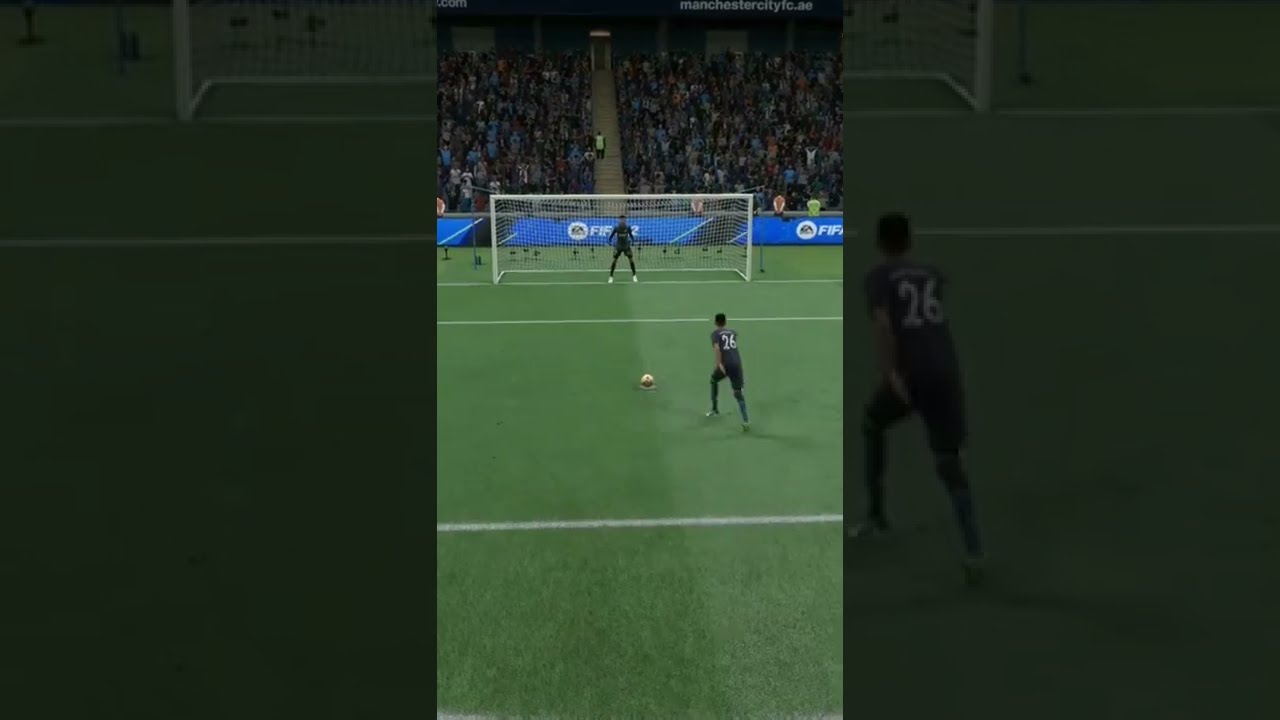The image is a horizontally rectangular, computer-generated scene that mimics a soccer match from a FIFA video game. It comprises three sections with the middle panel prominently displaying the action. In this central panel, the backdrop features a filled stadium with an audience and a visible staircase dividing the crowd. In front of this, there is a soccer goal with a goalie poised at the center. The focal point is a soccer player wearing a dark blue uniform with the number 26 in white on his back, preparing to take a penalty kick. The yellow ball is set in front of him on the green field marked with white lines, and he is just about to strike it.

Flanking the central action are two darkened sections that provide a slightly enlarged, shaded view of the same scene. The left section shows a part of the soccer field leading up to the goal post, while the right section provides a darkened glimpse of the soccer goal's right side and a portion of the field. Together, these sections frame the vivid action in the middle, emphasizing the anticipation of the penalty shot and creating a dramatic, immersive visual narrative.